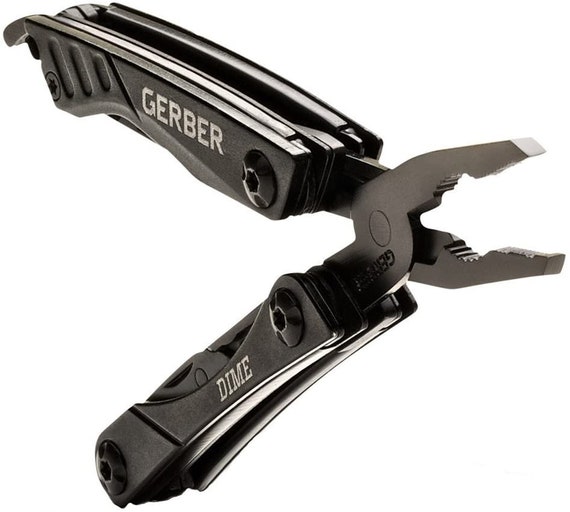This photograph showcases a highly detailed, zoomed-in image of a multi-use tool, prominently featuring a pair of pliers. The tool, possibly designed for an advertisement, is primarily dark gray in color with metallic overtones. It is open, with the blades positioned on the right side of the image. The tool's handles are notable for their intricate inner workings, visible on both the top handle, which is labeled “Gerber” in white text, and the bottom handle, which reads “Dime” in white text. These labels are clearly displayed on the dark gray handles. The pliers also seem to incorporate additional tools, including a flat-head and a Phillips screwdriver, though these are less prominently featured and somewhat difficult to discern. The entire background is a consistent white, providing a strong contrast that highlights the detailed design and screws bolted into the top and bottom of each handle.